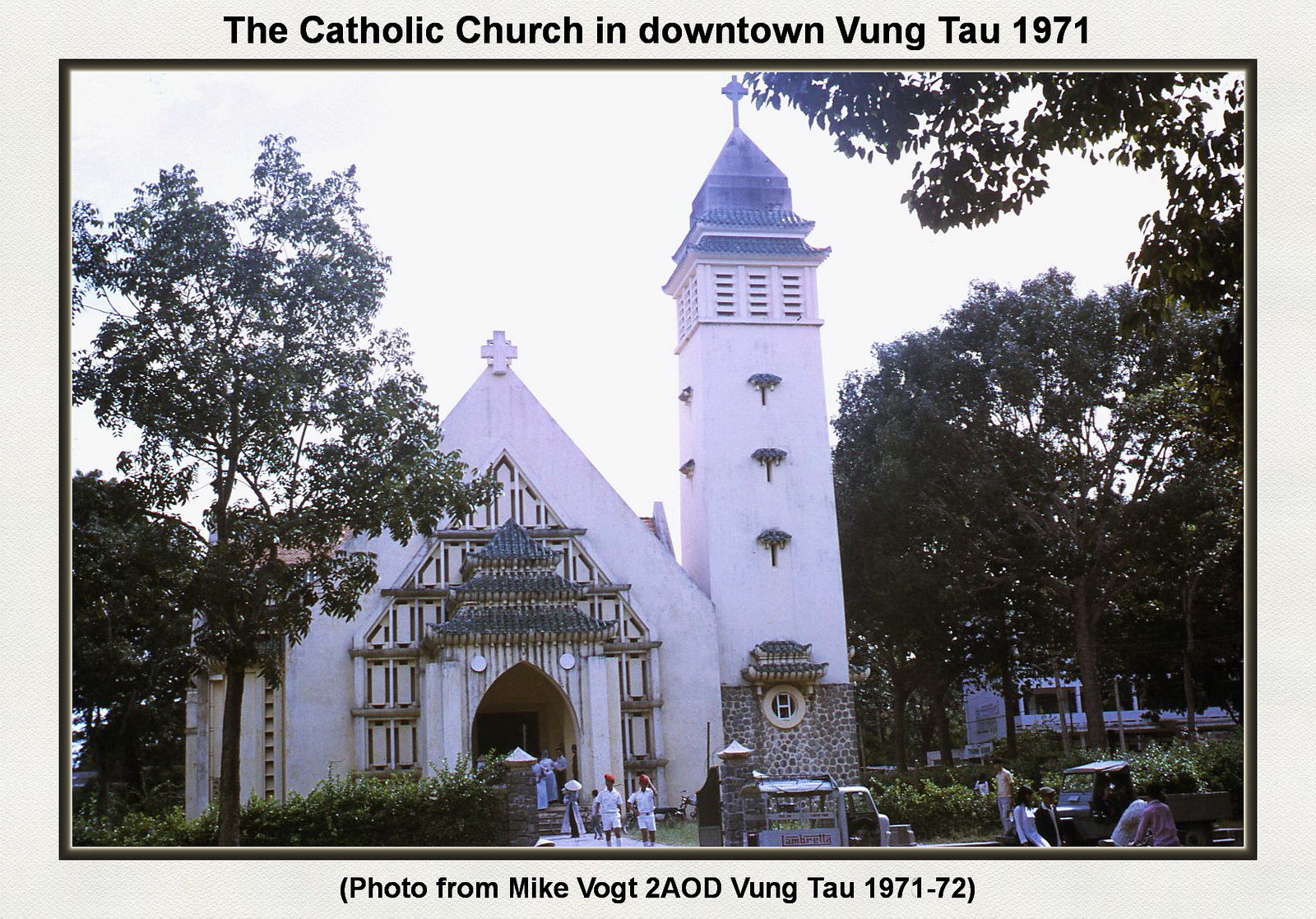The photograph depicts the facade of a white Catholic church in downtown Vung Tau, Vietnam, taken in 1971. The church's architectural features include an angled, pointy white facade with an arched roof, and intricate embellishments resembling three-tier shingles. To the right of the main body stands a tall tower crowned with a blue cross and a roof of the same blue color and texture. The foreground shows steps leading up to the entrance, with several people walking in and out of the church. Surrounding the church are tall trees with dark green leaves, framing the scene against a backdrop of a cloudy daytime sky. The image is bordered by a cream-colored frame, with black text at the top reading, "The Catholic Church in downtown Vung Tau 1971." Below that, in parentheses, it reads, "Photo from Mike Vogt to AOD Vung Tau 1971-72."